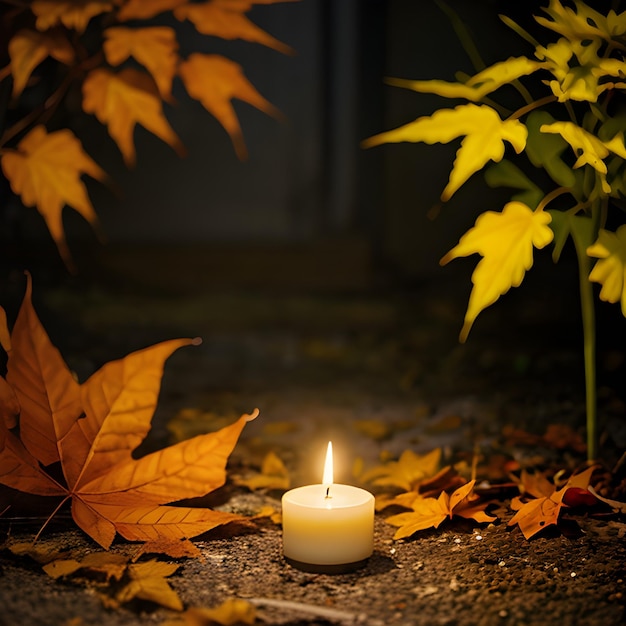This full-color, vertically rectangular photograph, staged outdoors at night using natural light, prominently features a small, lit white candle. Located at the center bottom of the image, the candle sits on brown dirt, its bright amber flame casting a warm light on its surroundings. Scattered around the candle are dead leaves in shades of yellow and orange, with some leaves positioned higher up, illuminated by the candle’s glow. The backdrop is softly blurred, revealing a white door nestled in the background, hinting at a nearby structure. Above the candle, thin branches adorned with yellow and orange leaves hang downwards from the upper left and right sides. The scene, void of people, animals, text, or distinct backgrounds, exudes a cozy, serene ambiance enhanced by the vibrant, glowing colors of the leaves and the lone candle.